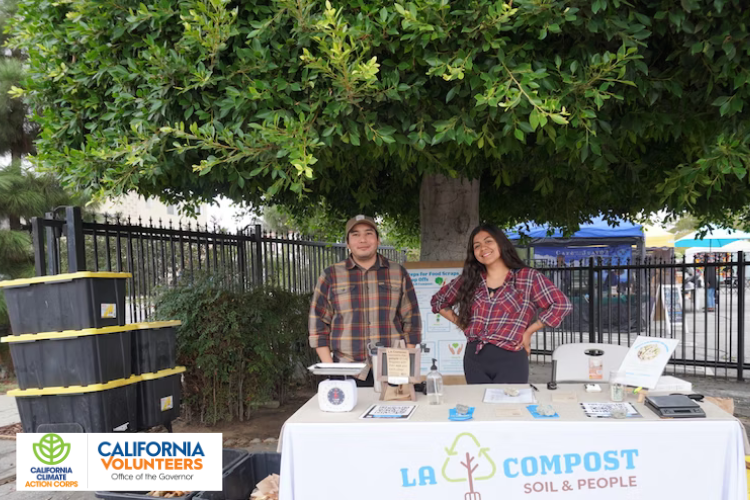The photograph, taken outdoors during the day with slight digital enhancement, showcases a square, full-color image with no border. At the bottom, a white banner reads "California Volunteers, Office of the Governor. California Climate Action Corps." The centerpiece of the image is a table covered with a white cloth that displays a green recycling logo and the text "LA Compost Soil and People." Behind the table stand a man and a woman, both in plaid shirts. The woman, on the right side, sports a red plaid shirt, long black hair, and a smile, with her arms on her waist. The man, on the left, wears a dark brown and slightly red plaid shirt, along with a baseball cap and a goatee. The background features a tall, bushy tree whose branches start a few feet above the couple, partially obscuring the sky. To the right of the table are black plastic boxes with white lids, stacked neatly, while to the left, there are additional containers with yellow tops. A black wrought-iron fence is visible, stretching across the yard. The entire scene conveys a community outreach event for LA Compost, with pamphlets and various materials displayed on the table.